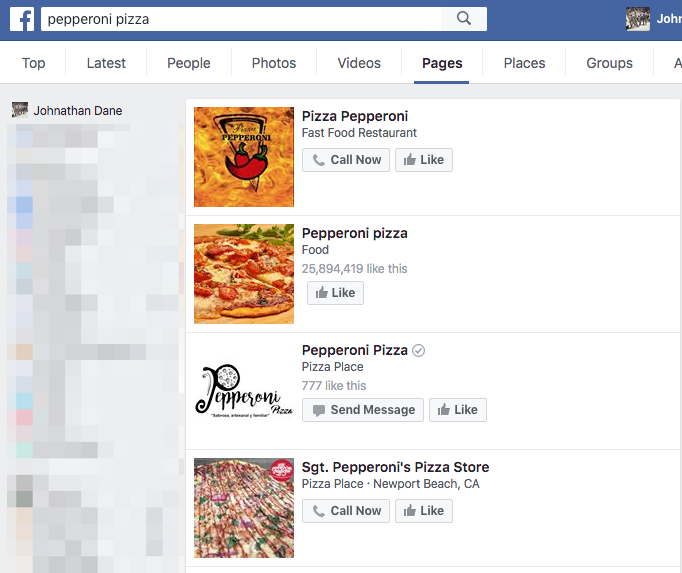The image captures a screenshot from Facebook showcasing various pizza places related to a search for "pepperoni pizza." In the upper-right corner, the user John is signed in, indicated by a thumbnail avatar next to his name. The Facebook interface highlights the "Pages" section, distinguished by bold black text with an underline beneath it. 

To the left, partially pixelated text reads "Jonathan Dane, D-A-N-E," likely anonymized for privacy reasons. Below, four different pizza business listings are displayed.

1. The first listing is for "Pizza Pepperoni," categorized as a fast-food restaurant, with options to "Call Now" or "Like." It features the restaurant's business emblem and a promotional image.

2. The second listing shows "Pepperoni Pizza," which is a generic thin-crust pizza with pepperoni on top. It boasts over 25 million likes and includes a "Like" button.

3. The third listing is another "Pepperoni Pizza," identified as a pizza place, with 777 likes, featuring options to "Send Message" or "Like."

4. The final listing is "Sergeant Pepperoni's Pizza Store" located in Newport Beach, California, with buttons to "Call Now" or "Like" and an image of their business establishment.

Each listing provides interactive options for users to engage with the respective businesses directly through Facebook.